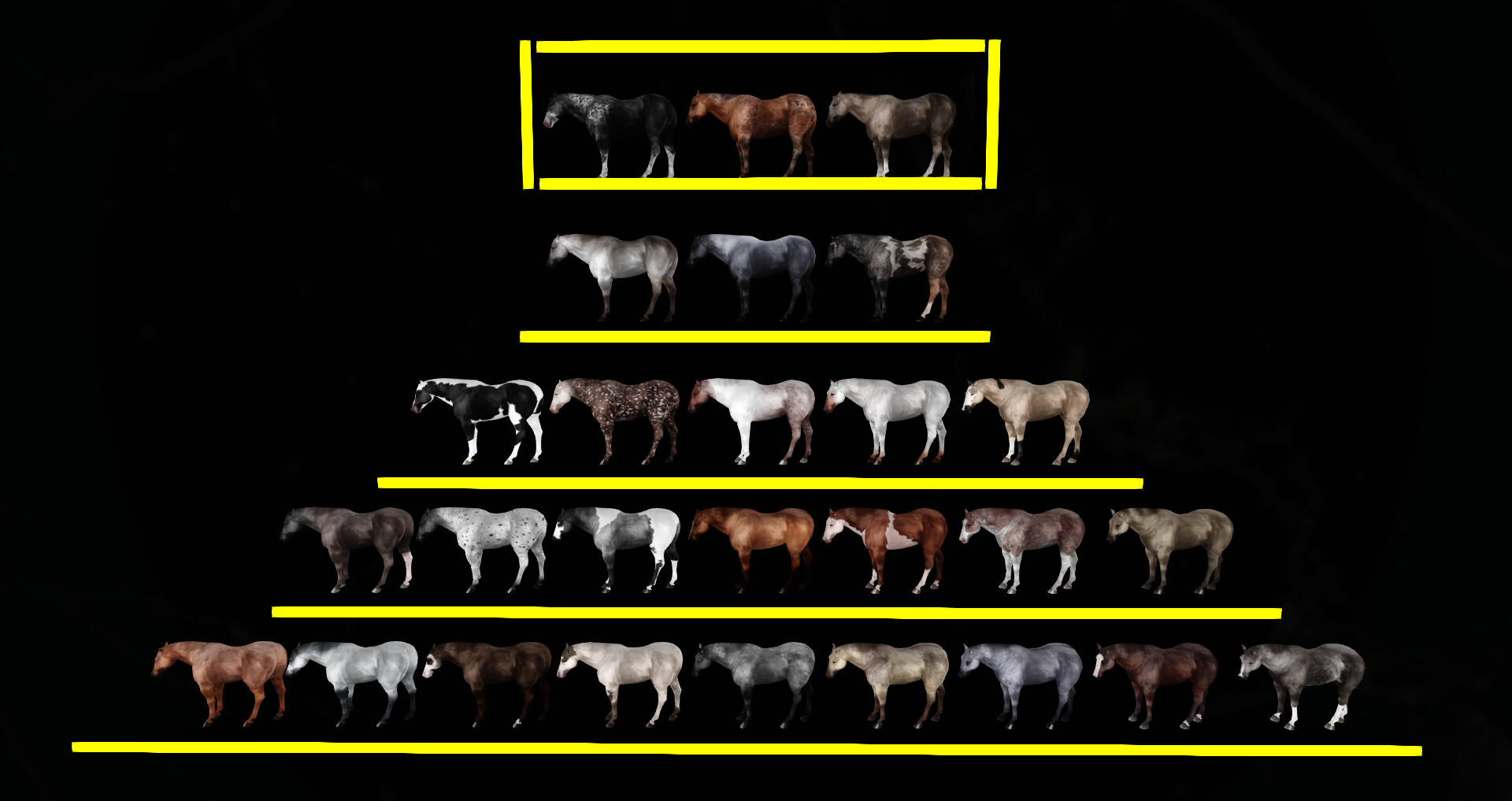This image features a black background adorned with multiple rows of horses, arranged in a symmetrical, triangular formation. At the top, a yellow-bordered box encloses three horses, which are colored black and white, brown, and brown and white. Below this, neatly organized rows are separated by yellow lines, which get progressively longer as they move downward, creating a pyramid shape. The highest visible row beneath the top box contains three horses: a white, a gray, and a brown one. Further down, each row increases in the number of horses—five in the next row, seven in the one following that, and nine in the bottom row. The horses display a variety of colors including brown, white, gray, black, and mixed patterns. All of them are uniformly facing to the left. The arrangement of yellow lines and the diverse coloration of the horses against the black background create a striking visual hierarchy.